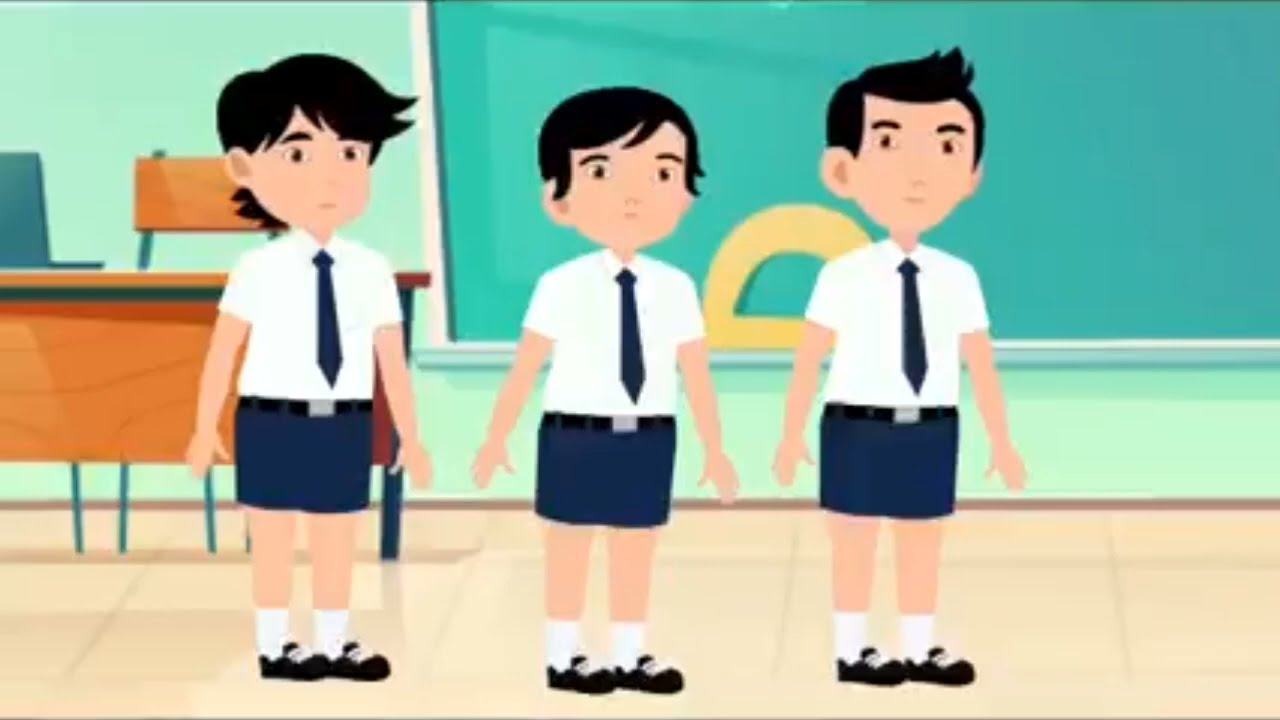The image is an illustration from a children's book or an animated video, depicting a cartoon classroom scene. It features three boys of lighter skin, possibly Asian descent, standing side-by-side in the middle of the frame and looking slightly off to the right. All three boys have black hair with varying short hairstyles and are dressed in identical school uniforms, consisting of white short-sleeved collared shirts, blue ties, blue shorts with black belts, white socks, and black shoes.

The background reveals a typical classroom setting with a large green chalkboard occupying the center to the right side of the frame. The chalkboard appears to have a protractor drawn on it. To the left side of the background, there is a wooden teacher's desk with a laptop open on it, accompanied by a chair. The walls of the classroom are painted a vivid lime green, and the floor is a contrasting yellow. Overall, the scene captures a moment of quiet and order in the school environment.